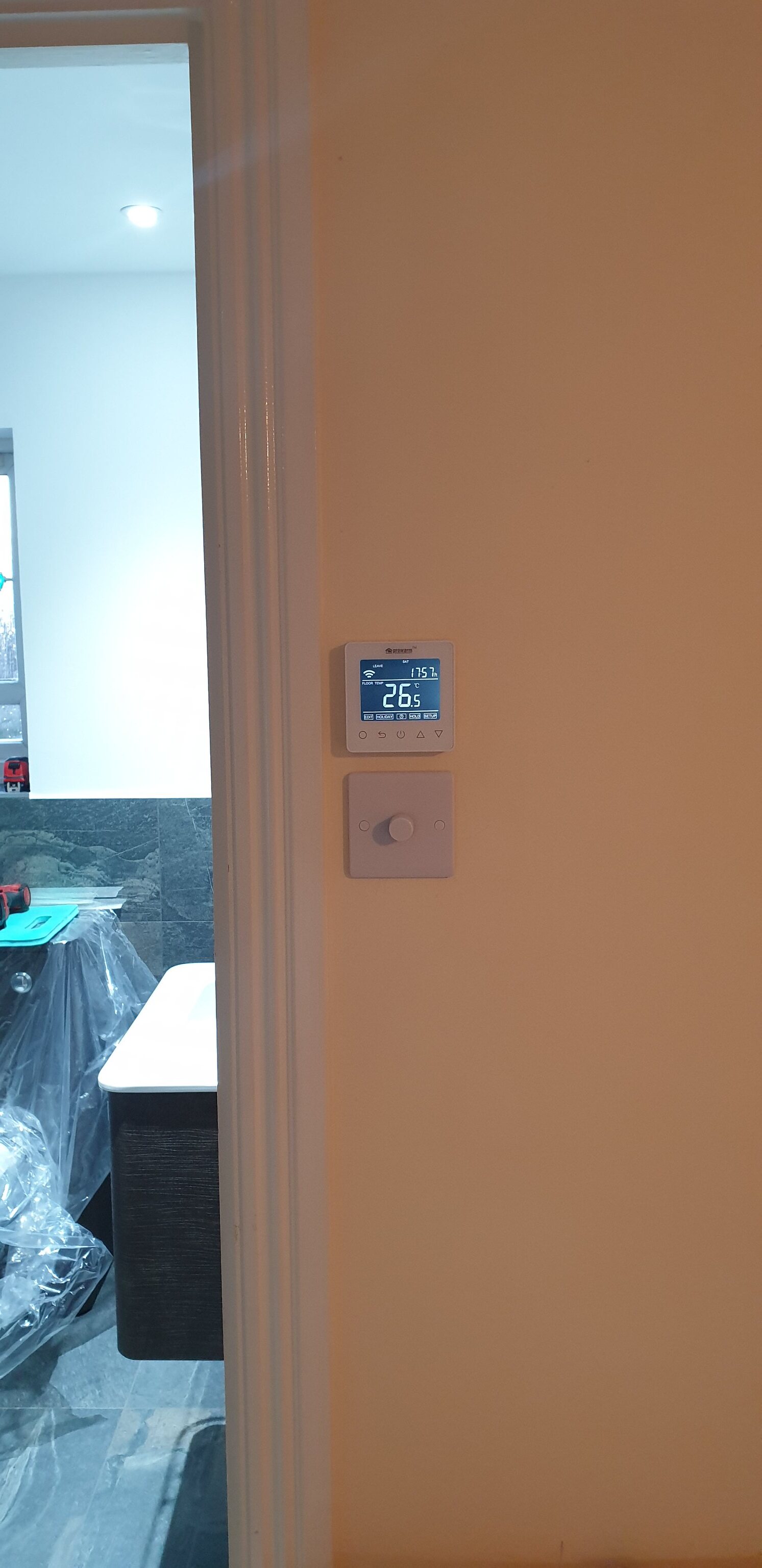The photograph captures the interior of a house, focusing on a wall and a doorway. The center-right of the image showcases a vertical door frame, adjacent to a peach-colored wall. Two notable objects adorn this wall: a digital thermostat displaying a temperature of 26°C and a time reading, albeit with small and unclear text likely indicating "11:57." Beneath the thermostat is a dimmer switch.

Through the doorway, a glimpse into the adjacent room reveals furnishings, many of which are covered in plastic. One uncovered item appears to be a desk or potentially a CPU unit, characterized by its tall, narrow black base and white top. The photographed scene suggests a space in the process of being organized or perhaps undergoing renovation.